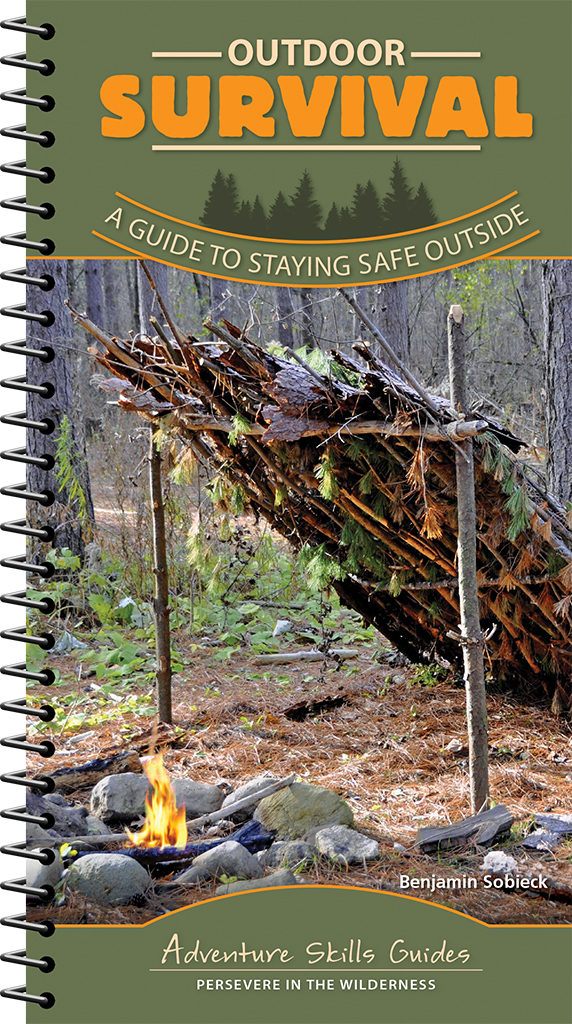This detailed product photo presents the cover of "The Outdoor Survival," a comprehensive guide written by Benjamin Sobiek. The spiral-bound, pocket-sized book makes it ideal for carrying in your jacket pocket while adventuring. Dominated by various shades of green, the cover features the title, "Outdoor Survival," prominently in orange lettering. The subtitle, "A Guide to Staying Safe Outside," further emphasizes the book's practical focus. Central to the cover is a photograph displaying a rustic, makeshift lean-to shelter constructed from branches and dead foliage, set in a woodland setting characterized by young, slender trees. In front of the shelter, there is a small fire encircled by stones, adding to the outdoor survival theme. The bottom of the cover reads, "Adventure Skills Guides - Persevere in the Wilderness," underscoring the book's purpose to equip readers with essential skills for wilderness survival.